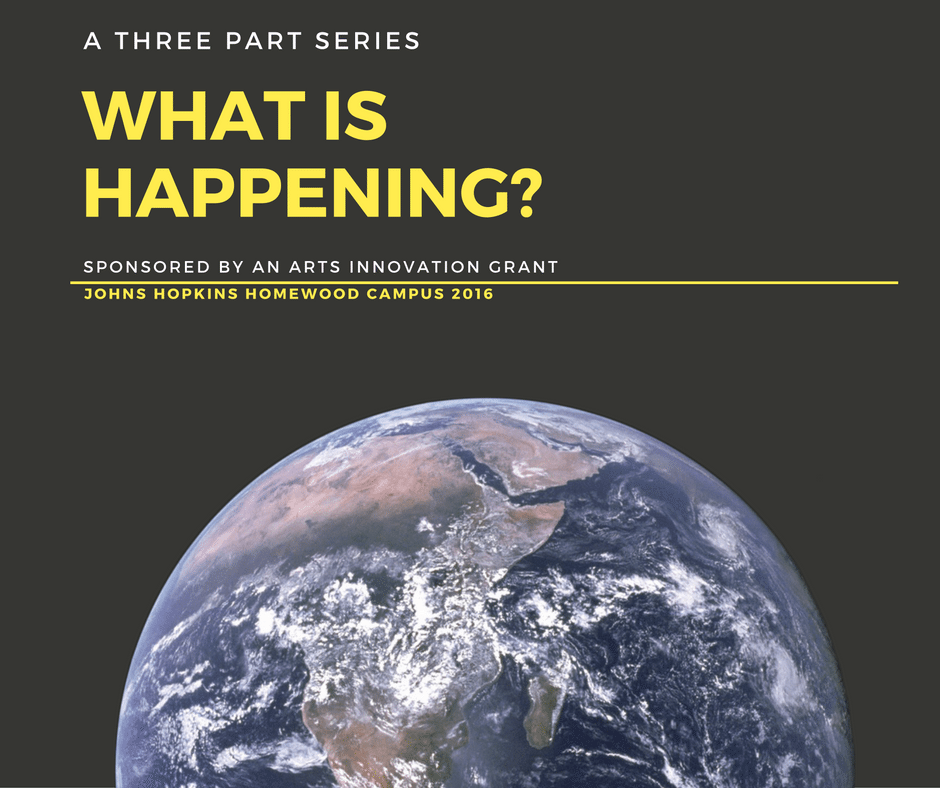Screenshot from a website announcing a three-part series. The background is black and slightly rectangular, possibly formatted for tablet display. The bottom half features a photographic image of the Earth from space, showing the top two-thirds of the planet. The text begins with "A THREE-PART SERIES" in white, all capital letters. Below that, in larger, bold yellow letters, it reads "WHAT IS HAPPENING." Further down, in white, all caps, it says "SPONSORED BY AN ARTS INNOVATION GRANT." A yellow line runs almost the full width of the image, with slight margins on the left and right. Beneath the line, in yellow, it states "JOHNS HOPKINS HOMEWOOD CAMPUS 2016." This series, hosted by Johns Hopkins, implies a focus on current events or issues, possibly involving the arts, though the specific theme isn't clearly stated.